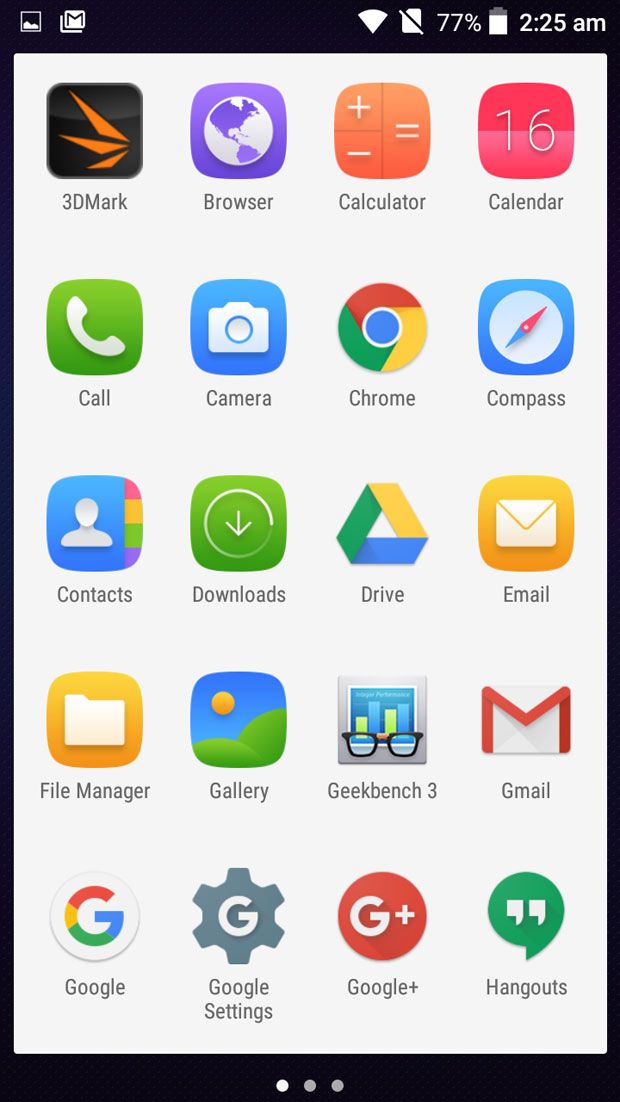The image features a smartphone screen with a distinctive black border encompassing all four sides. At the very top, the status bar displays the time as 2:25 A.M., a battery life of 77%, and full Wi-Fi connectivity, all set against a white background. Below this, there is a structured grid of application icons, arranged neatly into five rows of four icons each.

Each icon is accompanied by a descriptive label underneath. In the first row, the icons from left to right are for 3D Mark, Browser, Calculator, and Calendar. The second row features Call, Camera, Chrome, and Compass. The third row includes Contacts, Downloads, Drive, and Email. In the fourth row, the icons are for File Manager, Gallery, Geekbench 3, and Gmail. The fifth and final row displays icons for Google, Google Settings, Google Plus, and Hangouts.

At the very bottom of the screen, there are three small circles indicating the number of home screen pages. The circle on the left is highlighted in white, suggesting it is the current page, while the middle and right circles are in a light gray shade, indicating inactive pages.